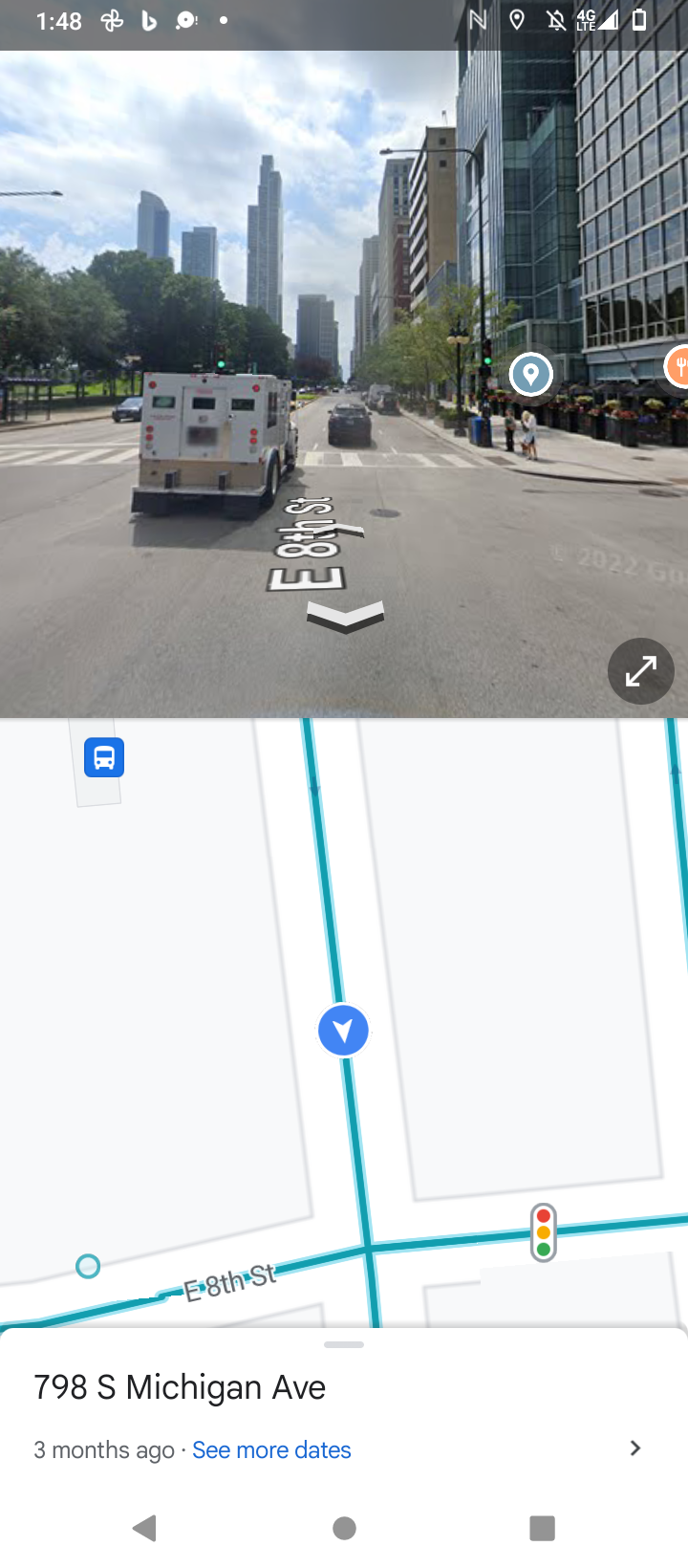The image is a tall, color screenshot from a cell phone displaying what appears to be Google Maps. At the top of the screen, the phone's status bar shows the time as 1:48, with a 4G LTE connection and a nearly depleted battery. Below the status bar, the screen is divided into two main sections. The top half portrays a first-person photograph of a city street labeled East 8th Street, featuring tall high-rise buildings with glass windows, a white truck, and several cars. You can also spot people standing on the sidewalk. The bottom half of the screen presents a simple, predominantly whitish or light gray map with turquoise-colored streets, depicting the route. The map indicates 798S Michigan Avenue and includes an icon resembling a teardrop pinpointing a location, as well as a blue line tracing the roadway. Additionally, there's a small traffic light icon visible. Overall, the image combines real-time visual navigation with a simplified map overlay.